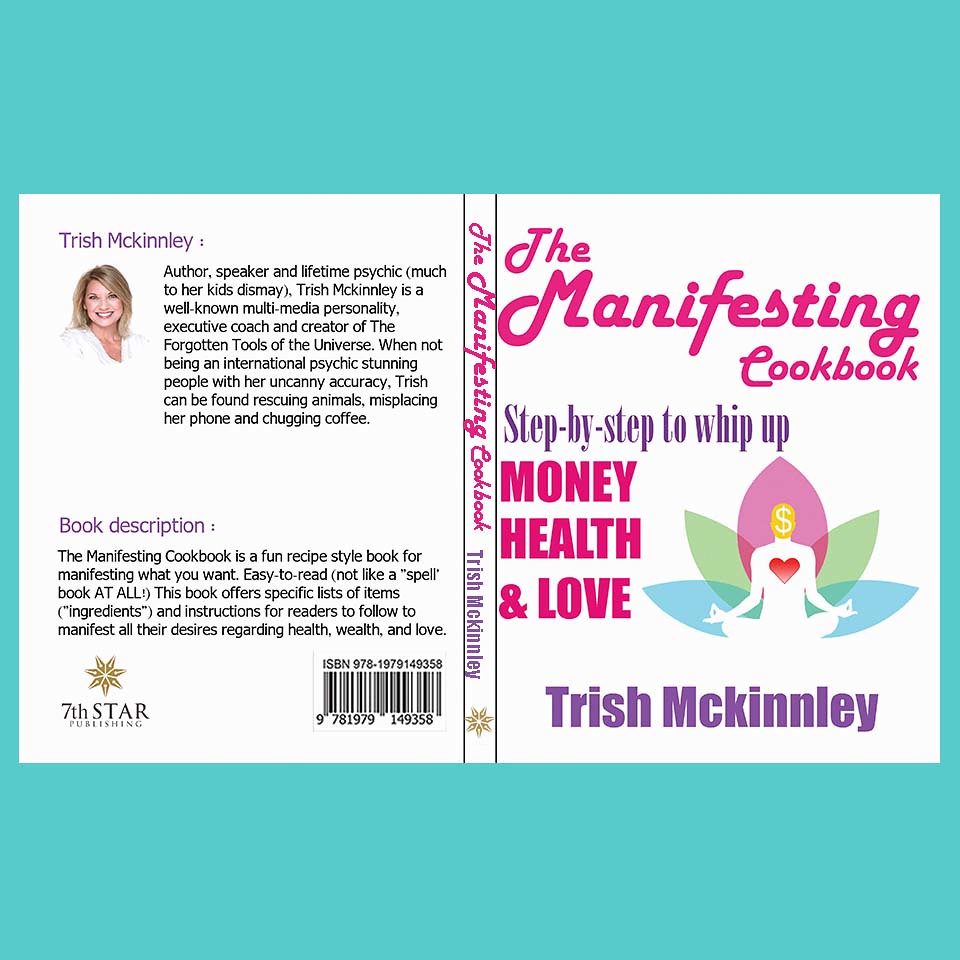The image presented is a detailed mock-up of a book cover, showcasing both the front and back along with the spine. The book, titled "The Manifesting Cookbook," features an ornamented font on its front cover (on the right) boldly displaying the title, "The Manifesting Cookbook: Step by Step to Whip Up Money, Health, and Love," with the author named Trish McKinley listed below. The front cover is adorned with an illustration of a person in a lotus position, mediating, with a heart symbol on their chest and a dollar sign over their head, surrounded by colorful oval shapes in blue, green, and red, creating a peacock-like effect.

The spine repeats the book's title, "The Manifesting Cookbook." On the back cover, there's a headshot of Trish McKinley, a woman in her early 40s with blonde hair and a light complexion, smiling warmly. The description next to her image introduces her as an "Author, Speaker, and Lifetime Psychic, Much to Her Kids' Dismay." It highlights her multifaceted career as a well-known multimedia personality, executive coach, and creator of the "Forgotten Tools of the Universe." A playful note mentions her activities like rescuing animals, misplacing her phone, and chugging coffee when she's not stunning people with her psychic accuracy.

Additionally, the back cover provides a concise description of the book itself. "The Manifesting Cookbook" is described as a fun, recipe-style guide for manifesting desires related to health, wealth, and love, with easy-to-read instructions, emphasizing that it is not akin to a typical spell book. At the bottom, flanked by a barcode and the logo for 7th Star Publishing, the book summary entices readers with the promise of specific lists of items, ingredients, and steps to help them achieve their dreams.